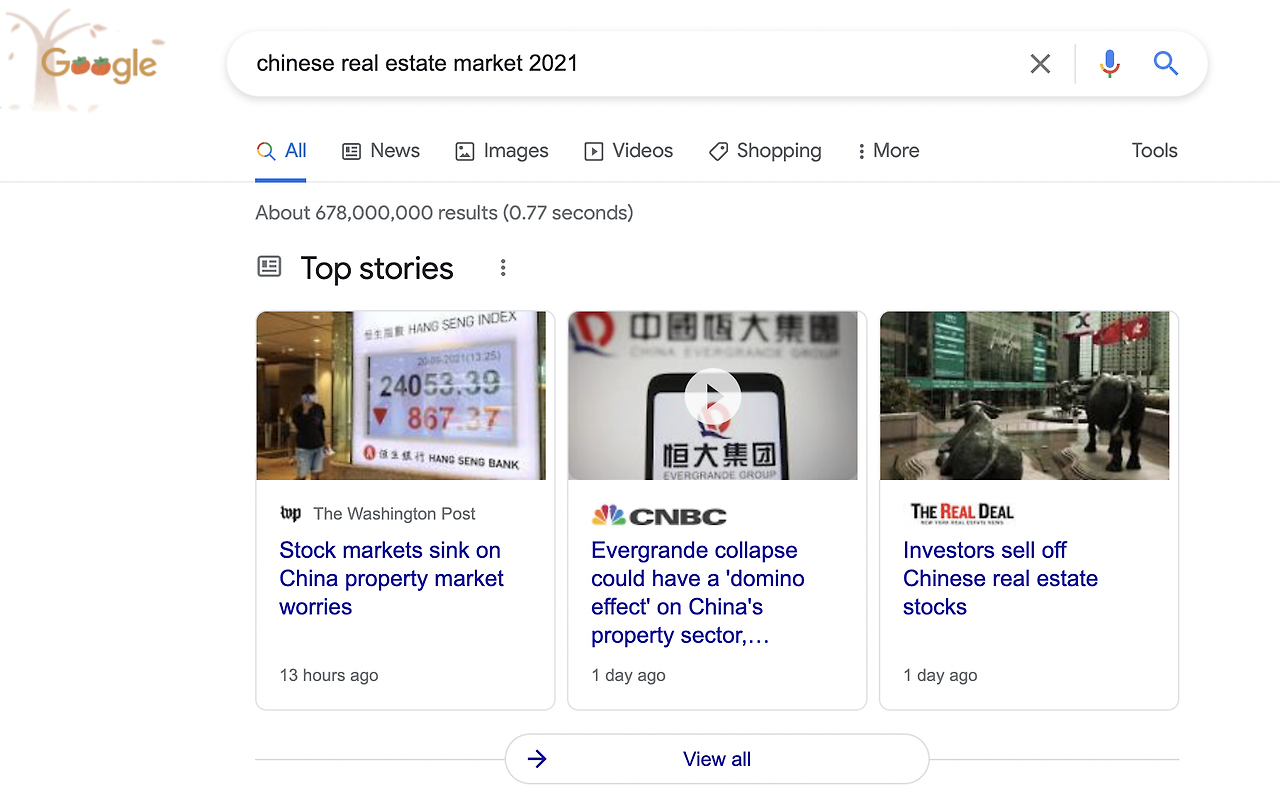In the image, a Google search results page is displayed, with several distinct features captured in detail. On the left side, the Google logo is prominently displayed in green, creatively featuring O's that resemble strawberries, accompanied by an artistic tree in the background with an orangey-brown color. 

On the right side, the search bar displays the query "Chinese real estate market 2021," indicating the subject of the search. Below the search bar, the usual navigation options "All," "News," "Images," "Videos," "Shopping," and "More" are visible, with the "All" tab selected.

The search results indicate approximately 60,678 million results found within 0.77 seconds. Below this information, a "Top stories" section showcases three main news stories about China's property market:

1. "Stock market sinks on China property market worries" with an accompanying image.
2. "Evergrande collapse could have a domino effect on China's property sector," sourced from CNBC, featuring a circular play icon suggesting it is a video.
3. "Investors sell off Chinese real estate stocks," sourced from The Real Deal.

These news stories are displayed with clickable blue links and brief descriptions. Below the middle news story, a large button labeled "View all" with a right-pointing arrow is evident, inviting further exploration. The overall design of the image includes a mostly white background with black and blue fonts, contributing to a clean and organized appearance.